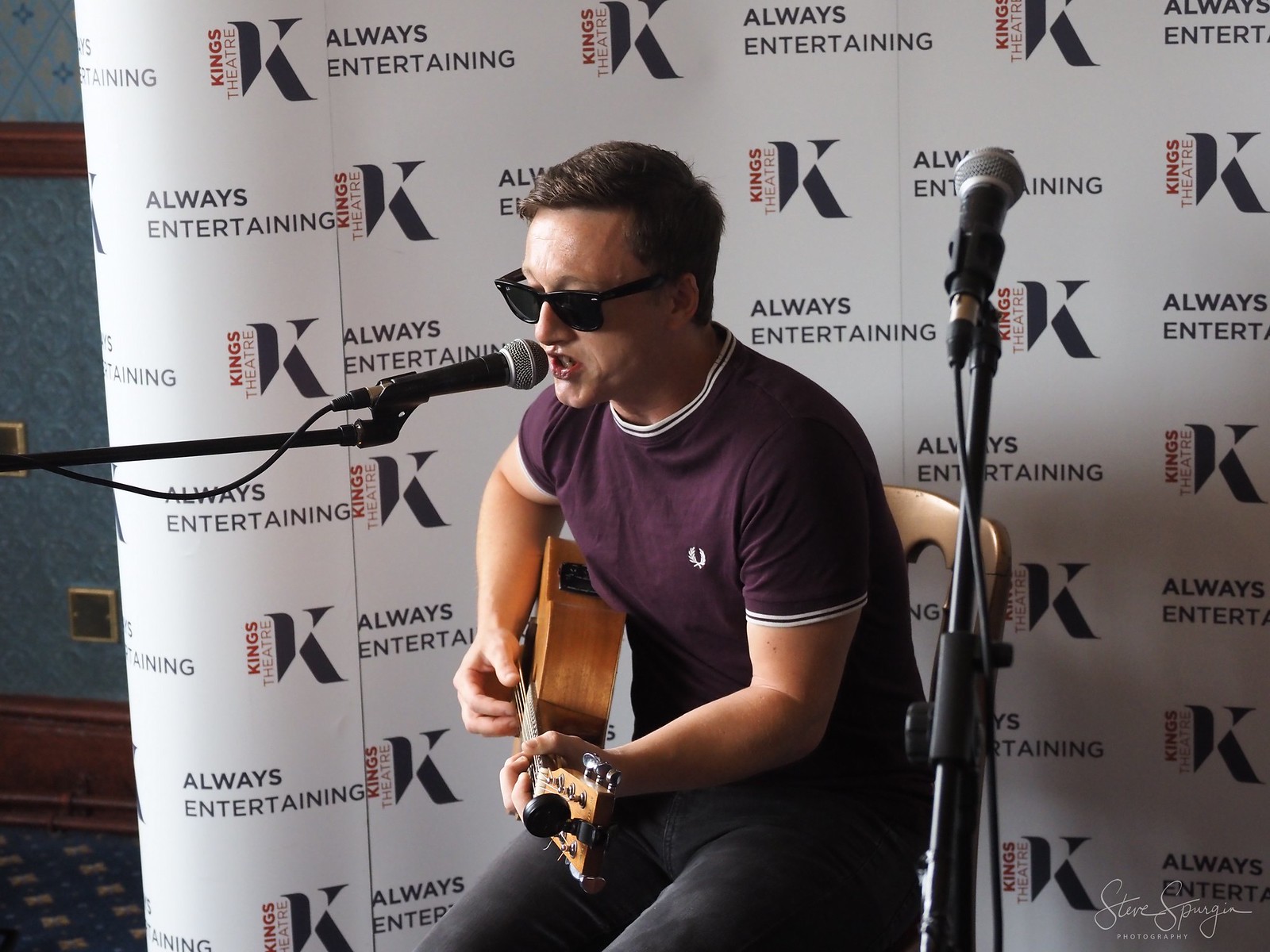A man is seated in a wooden chair in front of a press banner that features repeating logos of "King's Theatre: Always Entertaining." He is wearing a dark purple t-shirt with white trim, dark blue jeans, and dark sunglasses. The man is playing a wooden acoustic guitar and singing into a microphone positioned close to his mouth. The press banner behind him partially reveals a larger Kings Theatre logo featuring a large red "K" with the tagline "Always Entertaining." The photograph, rectangular in shape, also reveals some of the venue’s decor: a blue wallpapered wall with a wooden chair rail, high wooden baseboards, and patterned navy blue carpet with a tan design. Another microphone is set up to the right of him, standing at a higher level, yet no one else is visible in the frame, reinforcing the sense that he may be the sole performer, possibly at an open mic night or special event. The bottom right corner of the photograph carries the signature "Steve [surname] Photography."